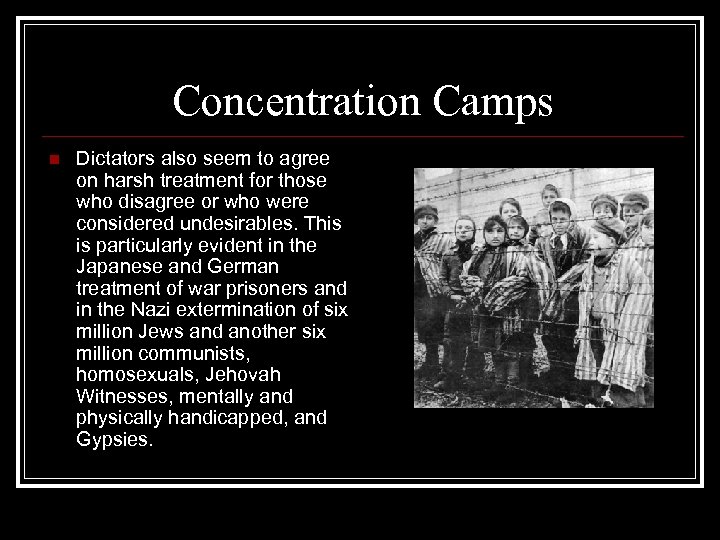The image appears to be a PowerPoint slide from a World War II presentation, focusing on concentration camps. Set against a solid black background, the slide includes a white-bordered rectangle containing both text and images. At the top, in white letters, it reads "Concentration Camps." On the left-hand side, there is a column of text preceded by a red bullet point, which states: "Dictators also seem to agree on harsh treatment for those who disagree or who were considered undesirables. This is particularly evident in the Japanese and German treatment of war prisoners and in the Nazi extermination of 6 million Jews and another 6 million communists, homosexuals, Jehovah's Witnesses, mentally and physically handicapped, and gypsies." To the right of this text is a poignant black-and-white photograph of children in a concentration camp, all dressed in tattered striped uniforms, standing behind barbed wire. The girls are seen wearing bonnets, while the boys have smaller caps. The stark imagery and detailed text highlight the grim reality and brutal treatment of people deemed undesirable by dictators during World War II.